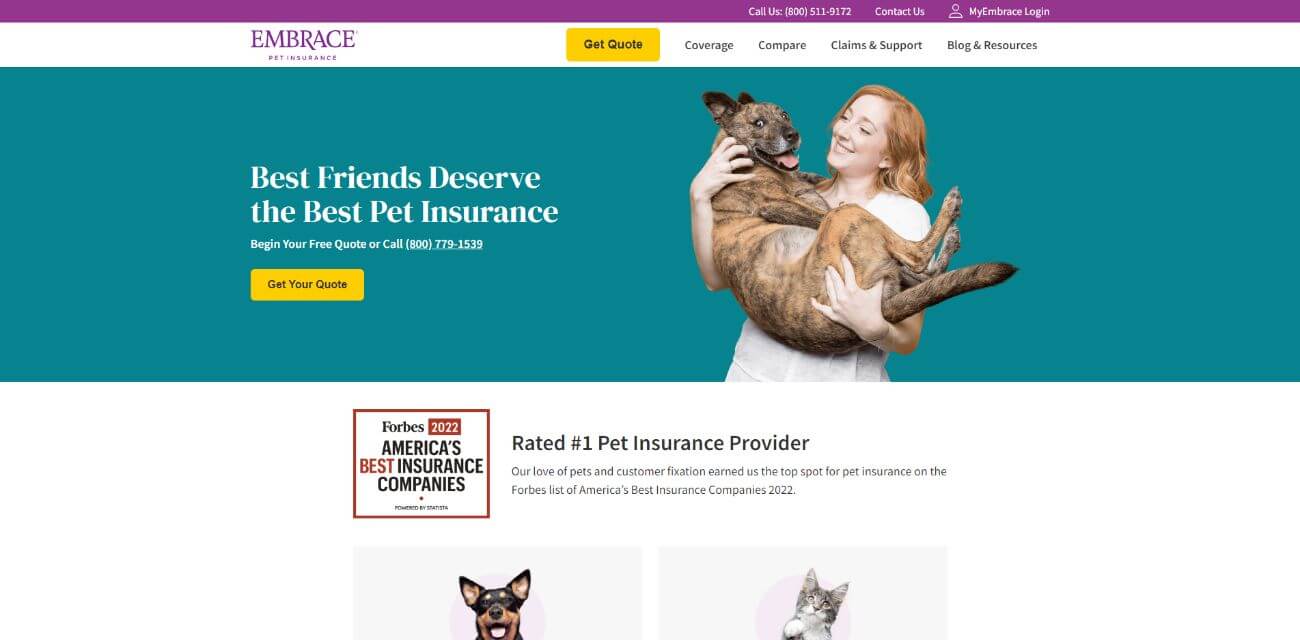The webpage features a prominent top navigation bar in a purple-pink hue. The right side of this bar displays the following white text: “Call Us: 800-855-511-9172” and “Contact Us.” Adjacent to these, there is a silhouette outline of an individual with the text, “My Embrace Login” beside it. 

Directly below this, a white horizontal bar spans the width of the page. On the left-hand side of this bar, the text “Embrace Pet Insurance” is displayed, with “Embrace” capitalized. To its right, there is a noticeable yellow button with black text that reads, “Get Quote.” Following this button are four navigational options: “Coverage,” “Compare,” “Claims and Support,” and “Blog and Resources.”

Beneath these elements, a banner with a blue background stretches across the page. On the left side of the banner, white text proclaims, “Best Friends Deserve the Best Pet Insurance. Begin your free quote or call 800-779-1539.” Below this text, a yellow button with black text states, “Get Your Quote.” 

To the right of the banner text, an image features a Caucasian woman with long, orangish-red hair, smiling and cradling her large dog, a brown dog with black stripes. The dog's mouth is open, revealing its tongue, and it has pointy ears, looking directly ahead. The woman is attired in a white shirt.

Beneath this banner is a red-outlined square with a white interior and black text stating, “Forbes 2022 America's Best Insurance Companies.” The “2022” in this square is highlighted in red text against a white background. The word “Best” is in red, while the rest remains black. To the right, additional text reads, “Rated Number One Pet Insurance Provider. Our love of pets and customer fixation earned us the top spot for pet insurance on the Forbes list of America's Best Insurance Companies 2022.”

Further down, there are two smaller squares. The one on the left showcases an image of a Doberman Pinscher with its mouth open, framed by a light pink circle. The square on the right displays a brown tabby cat with an extended paw, white paw, chest, and snout, also surrounded by a light pink circle.